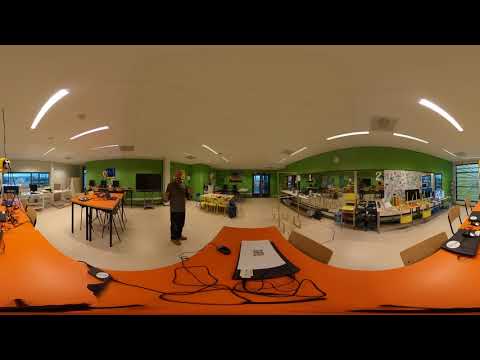This image is a panoramic shot taken with a wide-angle lens, depicting an indoor area likely to be a cafeteria or a public working lounge. The central focus is a long, rectangular orange table that appears wider due to distortion. Wooden chairs are neatly lined up along one side of the table. Placed centrally on the table is a laptop, with wires possibly indicating a charging station, making this area suitable for working or studying.

In the middle of the image stands a man dressed in a gray long-sleeved shirt and blue pants, possibly wearing a hat or a scarf. To the left of the man is another table that holds supplies, hinting at a classroom or workshop environment. In the background, the walls are painted lime green, and there are multiple sections likely meant for ordering food, seen as stations labeled "1" and "2". On the far right, there's an area that resembles a buffet or food trays, suggesting the functionality of a cafeteria. Additional areas with tables and computers are visible, enhancing the setting's multi-purpose scope. The ceiling is white with installed lights, overall contributing to a well-lit, functional space for both dining and working.